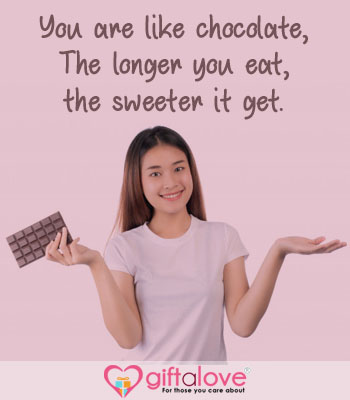The image is an advertisement for Gift A Love featuring a young woman, possibly Asian or Hispanic, with tan brown skin and long brunette hair that lightens towards the tips with a hint of red. She's wearing a light pink or pinkish-white shirt and is smiling while looking directly at the camera. Her pose is casual, with her shoulders shrugged and her palms facing outwards in a questioning gesture. In her right hand, she holds a chocolate bar composed of four by six dark brown squares. The background of the advertisement transitions from dark pink at the top to a lighter pink towards the bottom. The main text at the top reads, "You are like chocolate, the longer you eat, the sweeter it get," in a chocolate brown color, indicative of a possible typo. Below the photograph is the logo for Gift A Love, where "gift" and "love" are in pink, and "A" is in dark purple. Adjacent to the logo is a hot pink heart with a light pink center, featuring a wrapped present with a light blue body and an orange bow. At the bottom, the slogan "for those you care about" is printed in black.